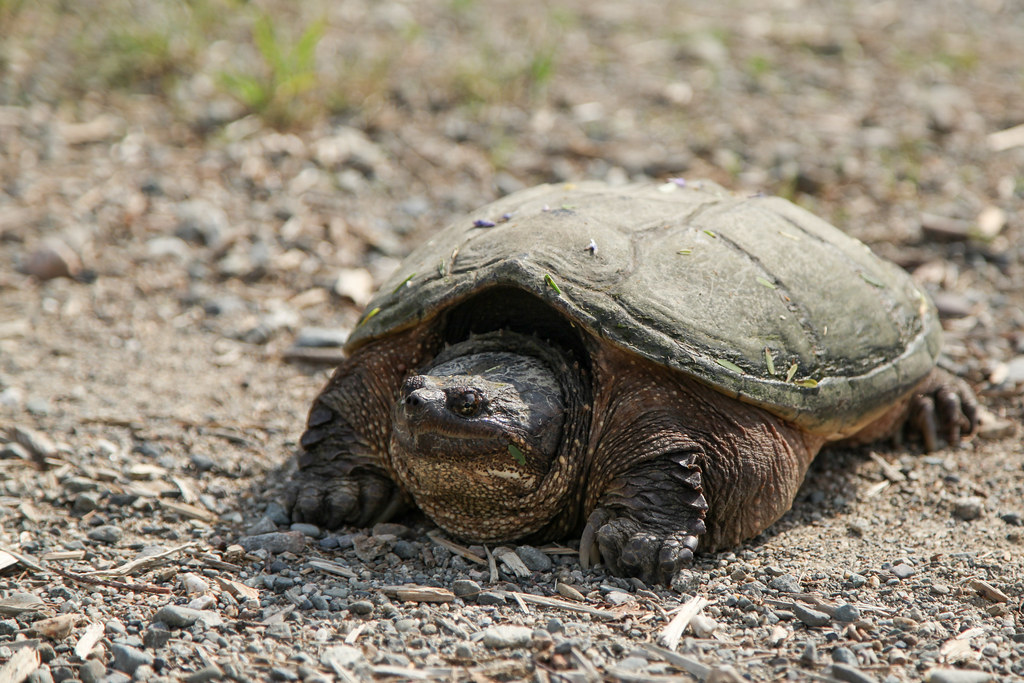This photo features a close-up, angled view of a large, old tortoise resting on a patch of dirt mixed with sand and gravel. The tortoise's textured skin and leathery, wrinkled neck speckled in lighter brown are prominently visible. Its head, mottled with black and brown eyes, is extended partway out of its greenish-brown and dust-covered shell, which also has scattered grass blades. The tortoise's rough, brown feet and long claws are emerging from beneath the shell. Bits of pebbles, branches, and grass are scattered across the dirt, adding to the scene's naturalistic feel. The blurred background highlights the tortoise as the central focus of the image.